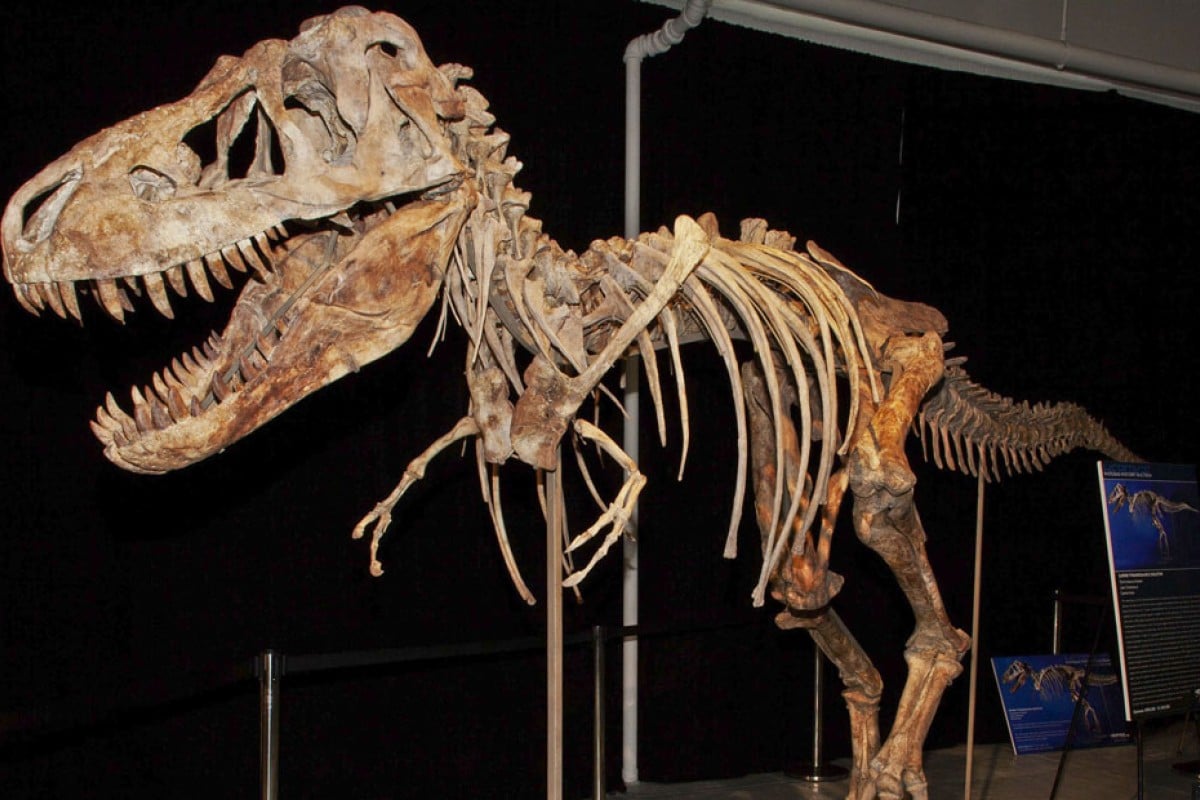The image is a detailed photograph taken indoors, showcasing a fossilized model of a Tyrannosaurus Rex skeleton prominently displayed in a museum exhibit. The T-Rex skeleton, which appears to be fully intact and cream-colored, dominates approximately 90% of the photograph. It is mounted in a dynamic pose as if running, with its mouth open, revealing sharp teeth, and its small arms positioned characteristically. The skeleton is secured by brownish-beige metal bars to keep it stable. Behind the fossil is a backdrop of black curtains, with a white pipe running vertically from the ceiling. In the lower right-hand corner of the image, there are two easels with dark blue posters. Each poster features an image of the T-Rex skeleton along with informational text about the exhibit. The overall setup creates a dramatic and educational display, emphasizing the grandeur and historical significance of the Tyrannosaurus Rex.